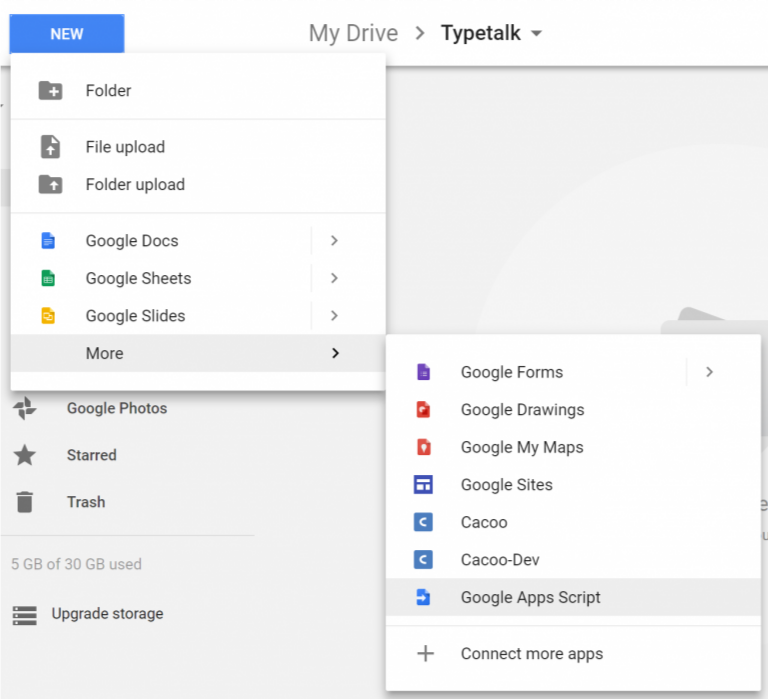The image displays the settings interface for Google Drive, meticulously organized into several categories. The top section features a blue header with scripts for "New," "My Drive," and "Type Talk." Below it, a column labeled "Folders" includes options for "File Upload," "Folder Upload," "Google Docs," "Google Sheets," "Google Slides," and "Google Photos." To the right, there's a segment featuring options like "Start," "Try," "5GB," and "30GB (Upgrade Storage)."

Additionally, there are several other components such as "Forums," "Purple Sheets," "Google Forms," "Google Drawings," "Google My Maps," "Google Sites," and "Kaiku," along with a specific reference to "Kaiku Dash 10." More advanced options listed include "Google Live Script" and "Kinect for Apps."

In the background, the interface is shaded in grey, listing items in seven rows sequentially numbered from 1 to 7. The entire layout appears to be dedicated to managing settings and various functionalities within Google Drive.